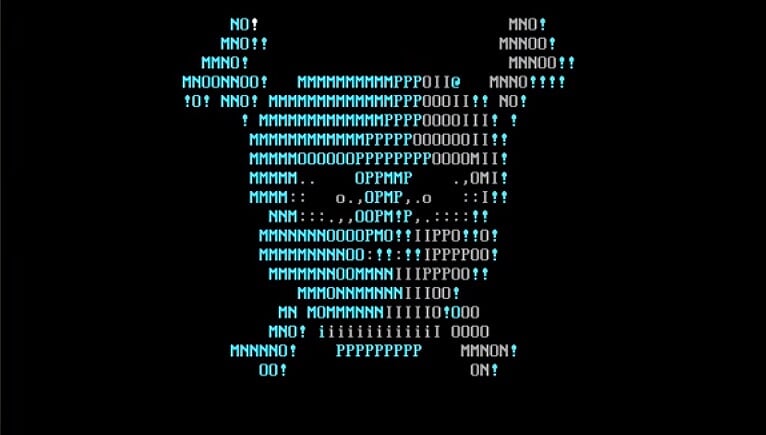This is a computer-generated image of a skull and crossbones on a solid black background. The skull and crossbones are intricately composed of the letters M, N, O, and P, as well as the numbers 1 and 0, exclamation points, semicolons, and commas. The design features two O's that effectively form the eye sockets, and the semicolons and commas are strategically placed around the eyes and nose to enhance the skull's features. The image shows a gradient in color: the left half of the skull is primarily composed of light blue letters, while the right half fades into gray. This detailed ASCII art creates a striking visual reminiscent of text-based graphics often seen in coding or on computer screens.